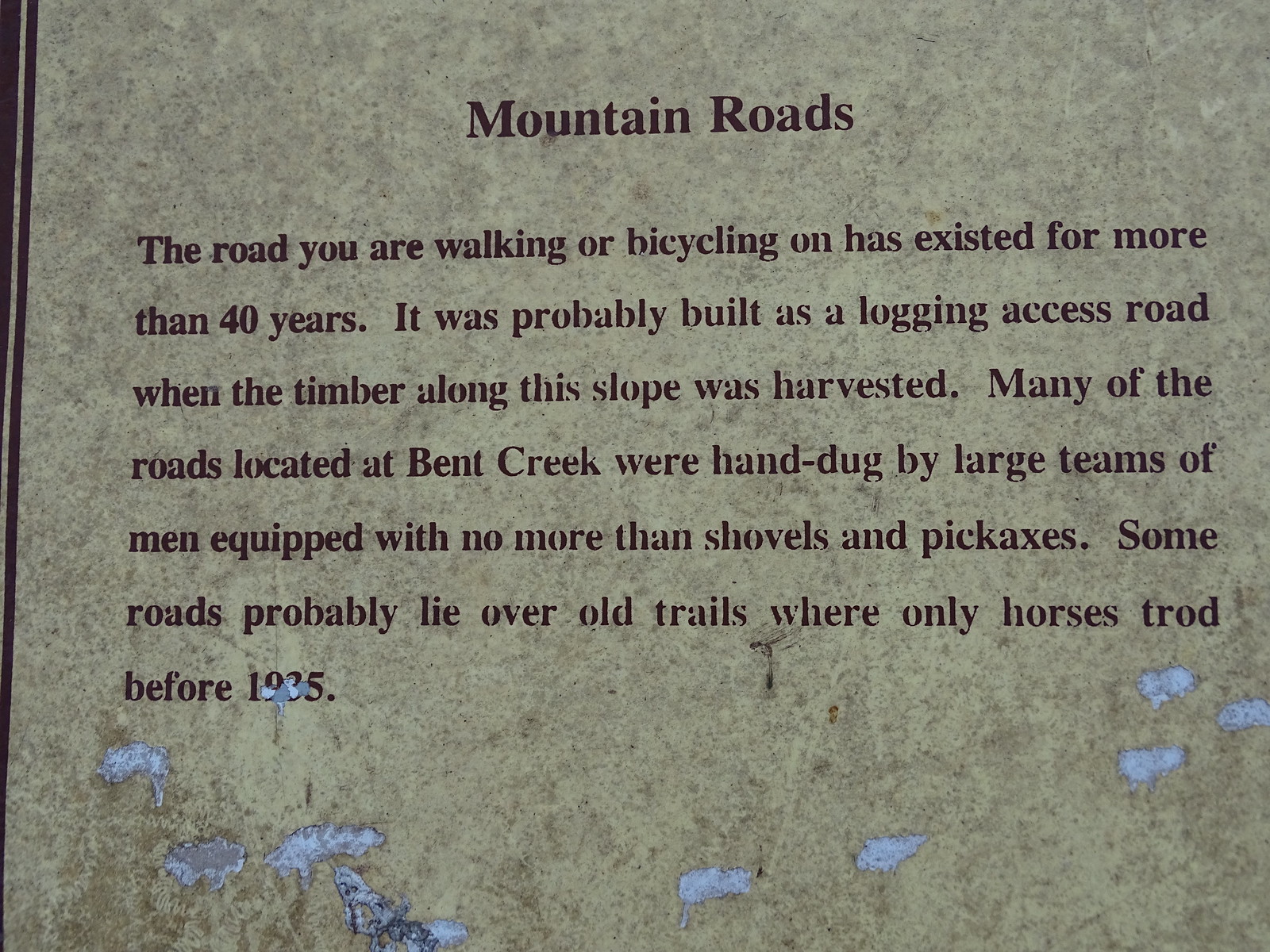The image is a photograph of a mountain road information sign with a greyish-brown background featuring white splotches at the bottom, partially obscuring the text. The sign is titled "Mountain Roads" in black text, followed by descriptive text in dark gray or black. It explains that the road you are walking or bicycling on has existed for over 40 years, likely originally built as a logging access road when timber was harvested along the slope. It further describes that many roads in Bent Creek were hand-dug by large teams of men using only shovels and pickaxes, and some roads may lie over older trails where only horses traveled before 1935.